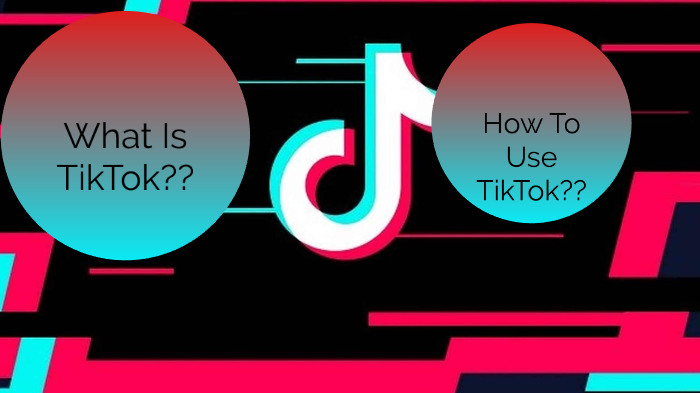Screenshot likely from a presentation or video about TikTok, set against a black background. The image features two prominent circles with an ombre coloring, transitioning from red at the top to a greenish-white at the bottom. The left circle, slightly off-centre vertically, contains the text "What is TikTok?", while the right circle, more centrally positioned near the top, reads "How to use TikTok?". In the middle of the image, the TikTok logo with its iconic white music note outlined in green and red is displayed. Below the logo are small, horizontal, thin lines in green and red, alongside thicker lines with right-angled protrusions near the bottom in red with green highlights. An additional similar element is partially visible behind the upper left circle. The text placement and overall design suggest a somewhat poorly formatted presentation on how to use TikTok.